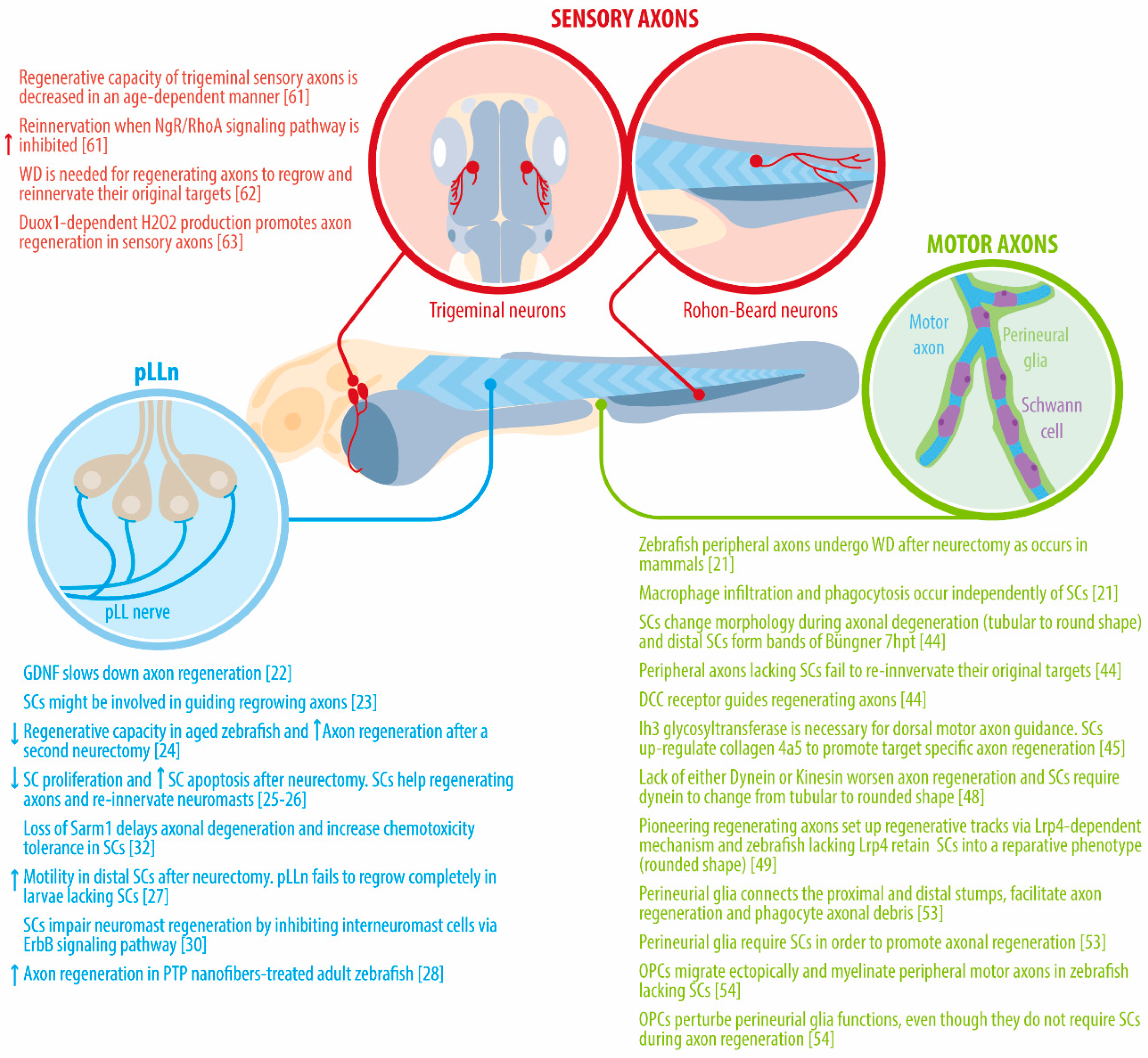This illustrated scientific drawing is a detailed educational tool designed for medical students and professionals, showcasing various types of neurons and axons. The diagram includes exploded views of structures such as sensory axons, trigeminal neurons, Rohan Beard neurons, and motor axons, emphasizing their functionality in sensory perception and motor function. Each neuron type is highlighted within color-coded circles that contain detailed illustrations and descriptive text. The red sections explain sensory axons and trigeminal neurons, emphasizing their role in touch and sensory feedback. The green sections detail the motor axons and their associated structures, such as Schwann cells, crucial for muscle movement and limb extension. The blue section illustrates the PLL nerve, with corresponding explanations. Furthermore, the diagram discusses the age-dependent decrease in the regenerative capacity of trigeminal sensory axons. The comprehensive annotations make this a valuable resource for understanding the complex structures and functions of neurons and axons.